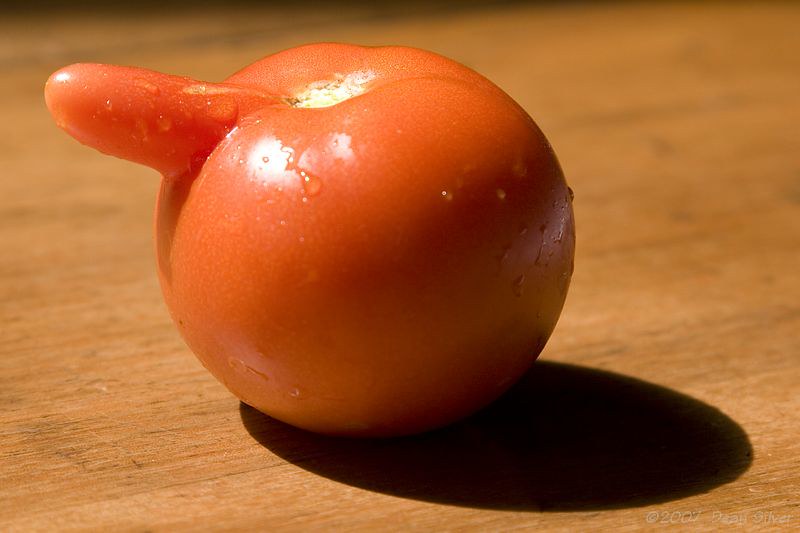The image features a close-up photograph of a deformed, red and orange tomato placed on a brown wooden tabletop. The well-lit scene casts a distinct black shadow diagonally towards the lower right corner, hinting that the light source is positioned from the upper left side. The tomato displays water droplets on its surface, suggesting it has either just been washed or has condensation from being refrigerated. At the top of the tomato, a peculiar growth emerges, resembling a finger or a small appendage, indicative of a genetic mutation. The deformation, with its white center and protruding node, adds an unusual and humorous aspect to the tomato’s appearance.